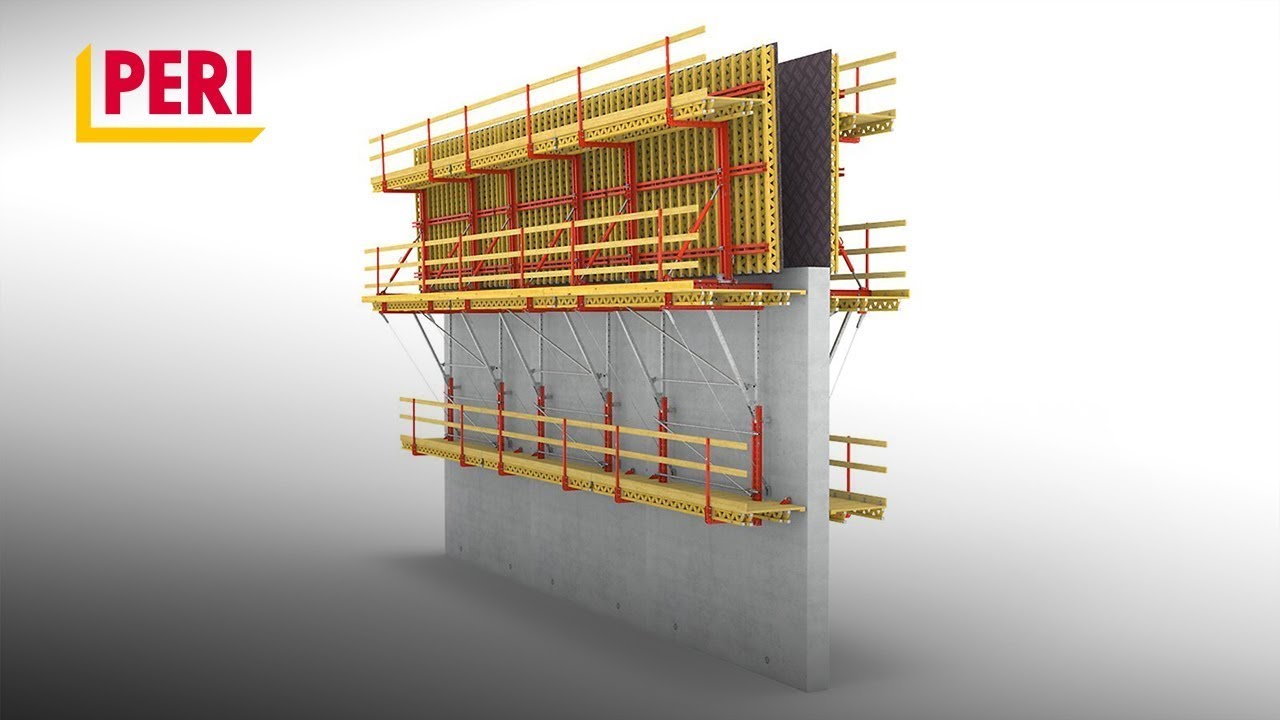This highly detailed color image, possibly a rendering, features a sophisticated scaffolding system set against a muted white and gray background. In the top left corner, there is a red logo spelling out "PERI." The main focus is a thin gray concrete wall, against which the scaffolding is mounted. The scaffolding itself is intricate, comprising a yellow, waffle-like grid structure that appears to be supported and reinforced by red beams and frames. Red posts mark the guardrails along the yellow platforms, adding to the complexity of the display. There's also a silver frame that seems to secure the entire setup directly to the concrete wall. The image conveys a technical and industrial aesthetic, likely intended for an advertisement of scaffolding equipment.